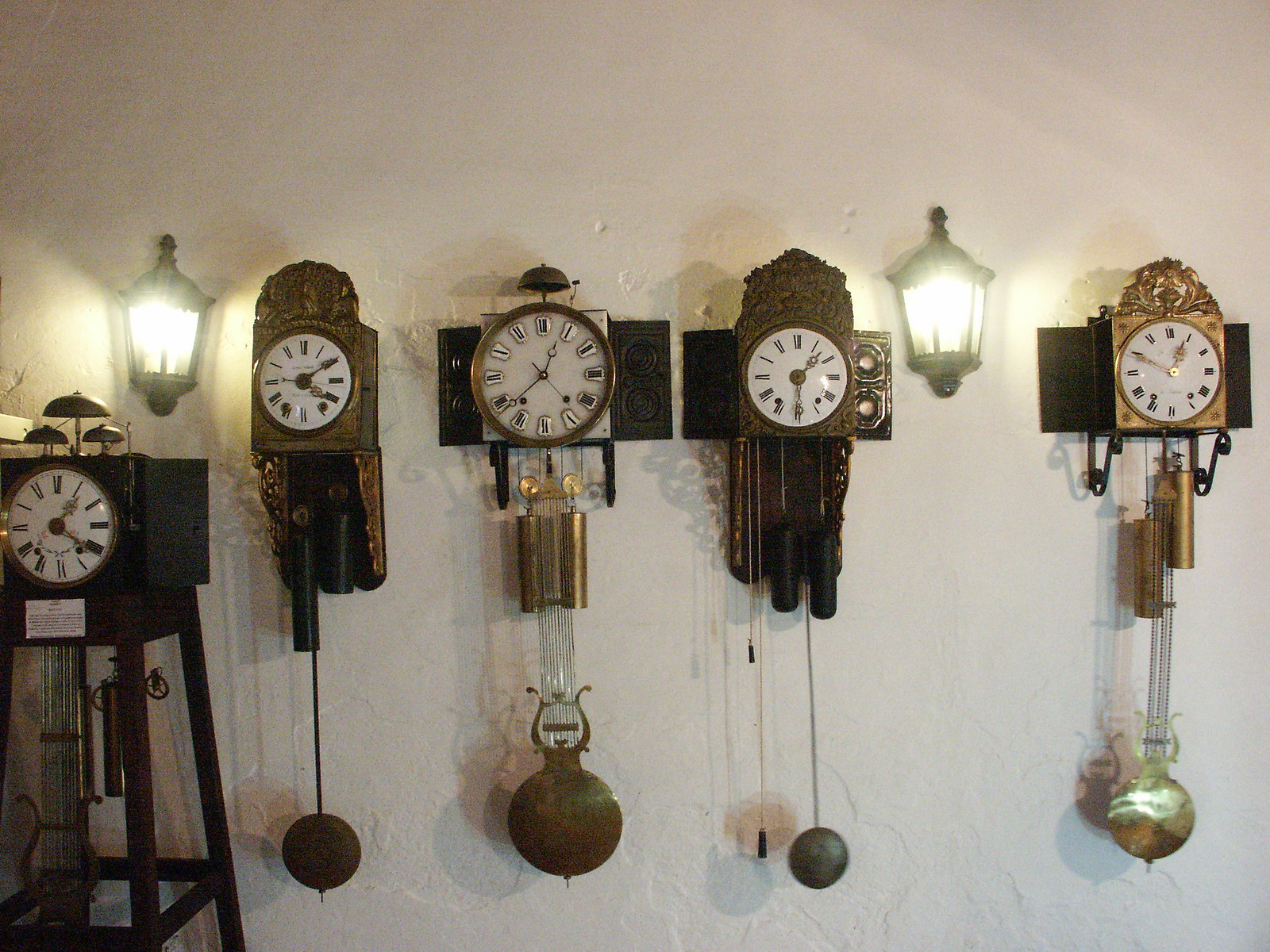This vibrant color photograph showcases five ornate, antique-style clocks hanging from a pristine white wall. Each clock features a white dial adorned with Roman numerals, and they all possess intricate design elements. Four of these clocks are perfectly aligned, suspended at the same height, while the fifth clock stands slightly lower on the far left. This leftmost clock resembles a deconstructed grandfather clock, elevated on tall legs with a central face, and embellished with hanging pendulums and bells, indicating it will chime at specific intervals. Beside the clocks, two glowing wall sconces add warm illumination, positioned symmetrically with one on either side of the arrangement. The clocks boast a rich, dark brown finish, with gold accents and hanging pendulums or chime-like pieces completing their picturesque, antique aesthetic.